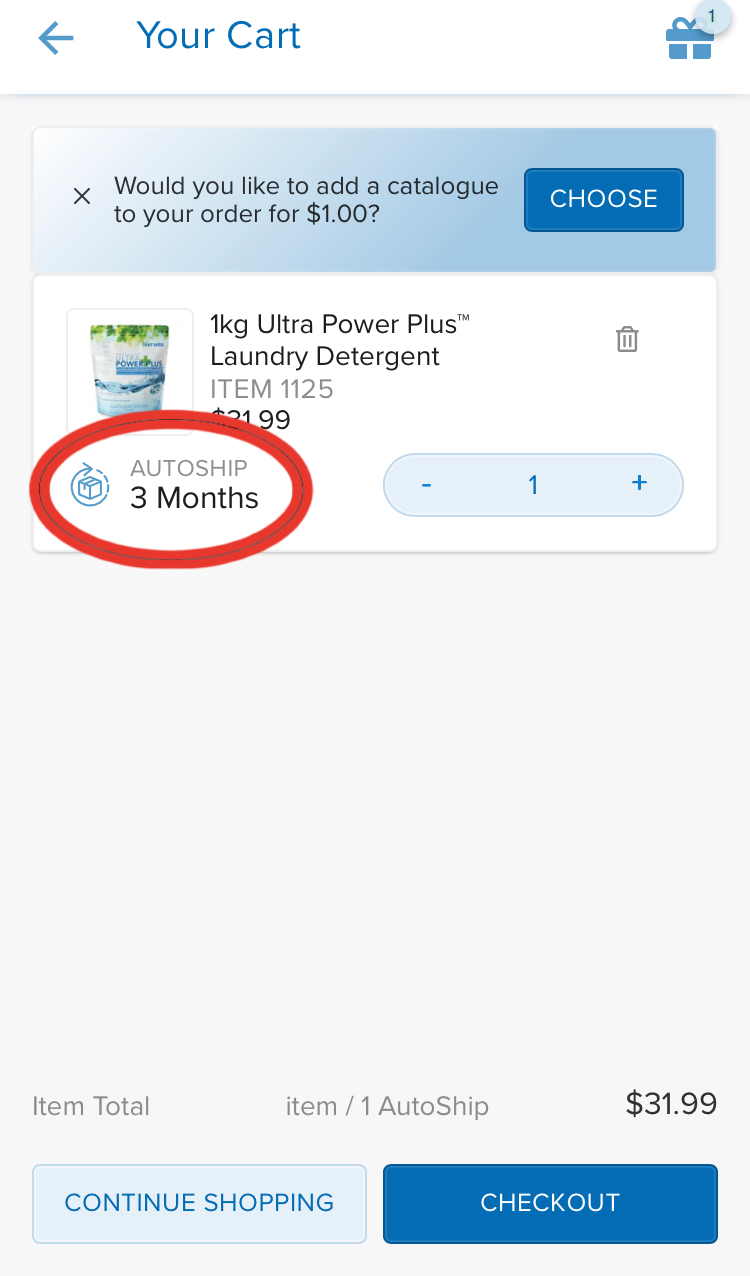This image is a screenshot from a desktop browser displaying a pop-up menu related to a shopping cart. The pop-up is primarily white and gray in appearance, with purple and blue accents. 

At the top-left corner of the pop-up, there is a white rectangle featuring a purple left-arrow icon followed by the words "Your Cart" in purple font. Adjacent to this text on the right, there is a purple present icon with a small light purple circle badge at the upper right, showing the number "1".

Beneath this section, there is a gray square containing a blue rectangle at the top, which includes a black "X" symbol. Next to it is a message in black text: "Would you like to add a catalog to your order for $1?" Below this message, a purple button with white text reads "Choose".

Further down, there is a large white rectangle displaying an image of a bag of detergent labeled "1kg Ultra Power Plus Laundry Detergent, item 1, 1, 2, 5". Overlapping the lower left corner of this product image is a large red oval. The text beside it reads "Auto ship three months". Towards the right of this product, a cursor is visible, indicating the user's interaction with the menu.

At the very bottom of the pop-up, in gray font, it displays "Item Total, Item / 1 Auto Ship," followed by "$31.99" in black font.

This comprehensive view suggests the user is considering their cart contents and supplemental options on a desktop e-commerce platform.